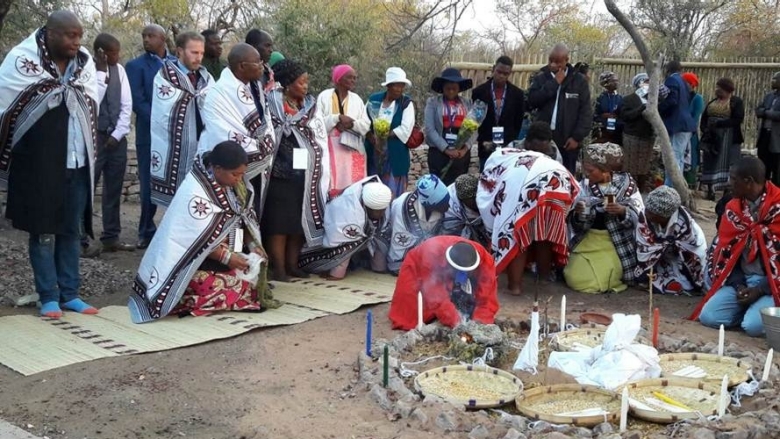The image captures an outdoor ceremony taking place on a clear day, set against a backdrop of a tree line. Central to the scene is a circle of stones with lit candles and circular flat baskets in the middle, emitting smoke. A man dressed in a red jacket with a white ring around his head kneels in front of the circle, seemingly starting a fire. Surrounding him in a half-circle formation are multiple men and women, some kneeling on mats or the dirt floor and others standing behind them. The participants wear draped blankets or sheets adorned with star patterns on the borders, featuring an eight-pointed star at each corner. A single white man is also present in the crowd. The scene has an air of ritualistic solemnity, possibly indicating a ceremonial or funeral event.